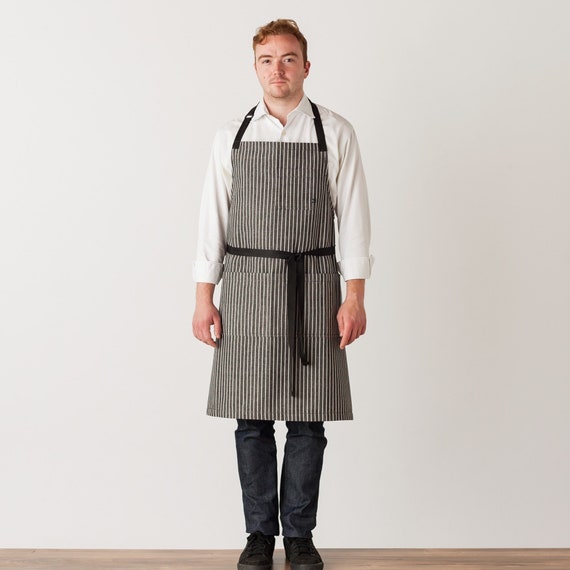The image features a young Caucasian man with short light brown to slightly reddish hair and a mustache with some stubble. He is posing against a white background wall, standing on dark tan wooden floors. He is dressed in a white long-sleeved shirt with the sleeves slightly rolled up, black denim jeans, and black shoes. Over his attire, he wears a black and white vertically striped apron, typical of a chef's uniform, with black straps around his neck and a wide black drawstring tied around his waist. The apron also features two pockets at the waist. The lighting in the picture appears diffused, coming from the right side and softly illuminating the subject. The man is looking directly at the camera, striking a composed pose.